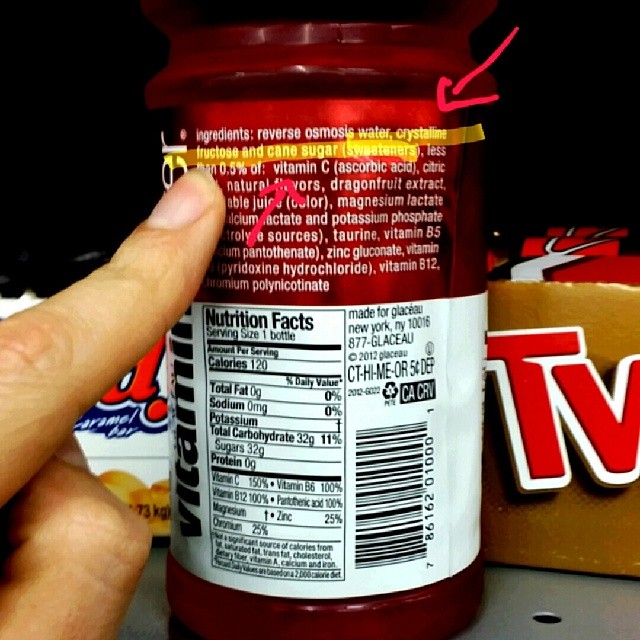Close-up photograph of the back of a red vitamin water bottle with the nutrition fact label prominently visible on the lower half, which is in white. A person's index finger, belonging to a white individual, is pointing to a highlighted section of the ingredients list. This section, highlighted in yellow, lists ingredients including reverse osmosis water, crystalline fructose, and cane sugar, with additional ingredients like vitamin C (ascorbic acid), citric acid, natural flavors, dragon fruit extract, and magnesium lactate. Two simple digital arrows are added to the image, one pointing diagonally from the right and another from the lower left toward the highlighted ingredients. In the background, shelves and items such as Twix and Payday candy bars are visible. The label indicates various nutritional facts: 120 calories per serving, 0 grams of total fat, 0 grams of sodium, 32 grams of total carbohydrates (11% daily value), 32 grams of sugars, and 0 grams of protein. The bottle also lists 150% of daily vitamin C, 100% of daily vitamin B6 and B12, 25% daily zinc, and includes a phone number for Glaceau in New York, among other manufacturing details. The upper portion of the background is black, and in the lower right corner, red letters "TV" are visible on the side of a cardboard box.